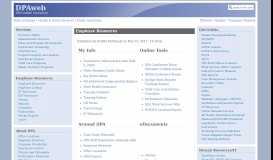The image depicts a small section of a website, with elements that are difficult to discern clearly due to its diminutive size. In its top left corner, there appears to be some text resembling "TIPAWELS," though the exact wording is ambiguous. A blue horizontal bar runs across the top, intersected by various shades of blue and a distinctive white swirl or swish in the center.

In the upper right corner of the website, there is a search bar. Below the blue bar, a narrow gray strip spans the page, containing listings under four different categories. The first three categories have text underneath them, whereas the fourth category remains empty.

On the left side of the webpage, there are three blue boxes, each denoted by its own heading. On the right side, there is one large blue box filled with numerous items listed within it. Beneath this large box is a small, shallow box with two visible items written in blue. It appears that this part of the website might be cut off, suggesting that one would need to scroll to view the full content of this section.